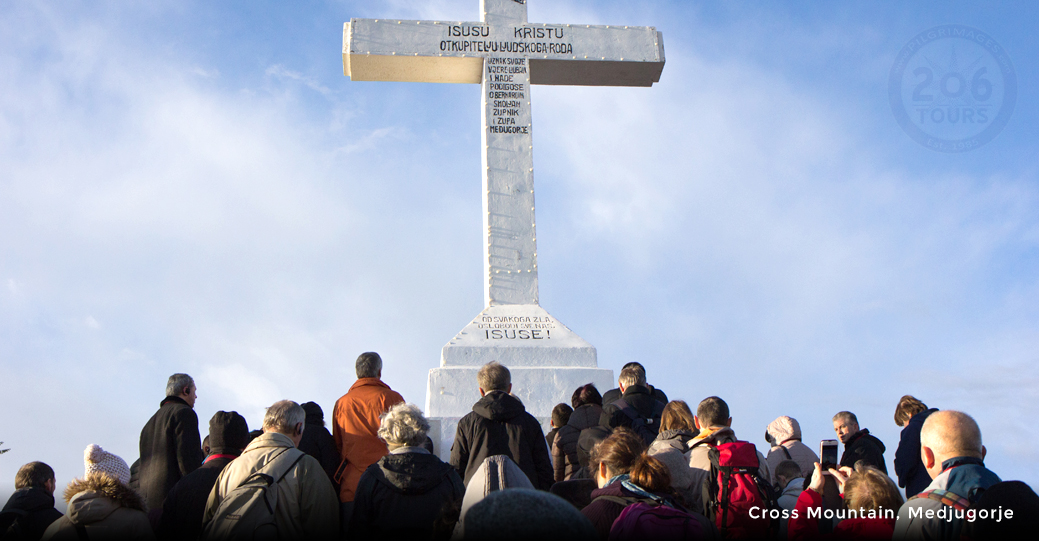The image captures a group of at least 25 people gathered reverently at the base of a large white stone cross atop Cross Mountain in Medjugorje. Bearing the watermark "206 Tourists," the photograph clearly labels the location in the bottom right corner. The cross, set against a vivid blue sky with wispy white clouds, prominently displays the words "Isusu Kristu" and additional text, presumably in Bosnian or Serbian, along its base. The scene features a diverse group of tourists, some kneeling and others standing intently, many of whom are taking pictures or holding backpacks. They are all dressed warmly in light jackets, indicating a possibly cool climate. The setting exudes a solemn and contemplative atmosphere as the visitors engage with the significant religious symbol before them.